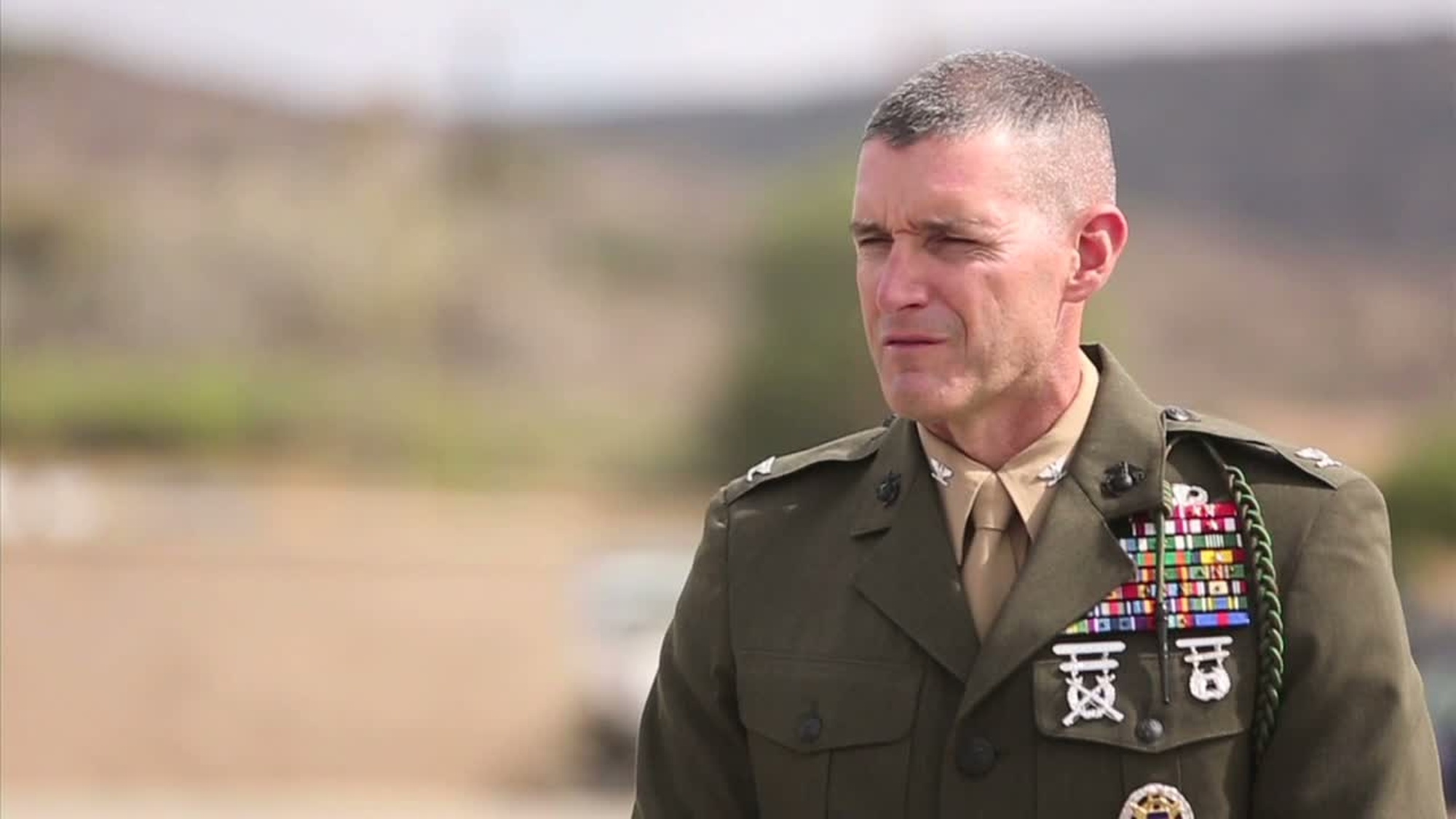In this color photograph, a man in military dress stands slightly to the right, looking to the left with a concerned expression, possibly in his late 30s to mid-40s. He has a very short crew cut hairstyle that is grayish-black and is clean-shaven. He squints as though it is sunny and hot. He wears a dark green, double-breasted military jacket adorned with numerous decorations, including eight rows of colorful bars, two pins, and a star encircled beneath his breast pocket. His uniform includes a beige shirt and tie underneath the jacket. The blurred background suggests a natural landscape with dry mountains and trees, adding to the focus on the solitary figure of the man in the photograph. There is no writing, and no other people or animals are visible in the image.